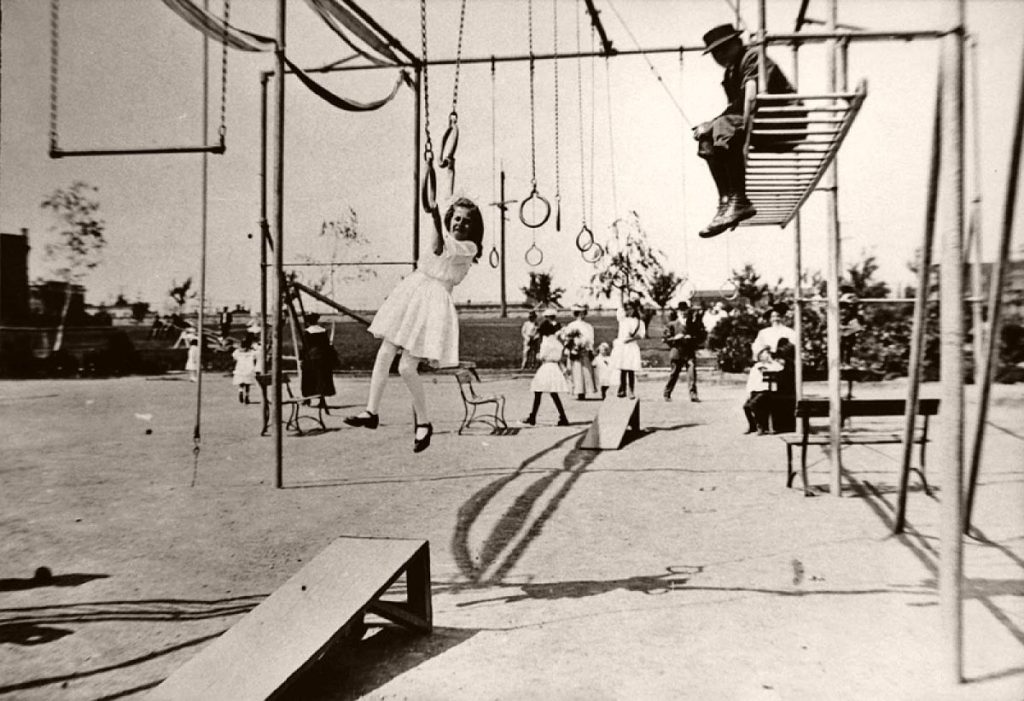In this detailed black-and-white image, we see a vintage playground bustling with activity. The large, iron-pipe play structures dominate the scene, featuring monkey bars that stretch from the foreground to the background, and rings hanging on chains, evoking an old-fashioned jungle gym setup. At the center of attention, a young girl in a white A-line dress, black Mary Jane shoes, and white tights is captured mid-swing on the rings, with one arm gripping each ring as she propels herself forward. To the right of the image, a man wearing a fedora and possibly a trench coat is seated atop the traditional monkey bars, attentively watching the children play below.

The background reveals a playground teeming with other children engaging with various equipment such as walking beams and possibly slides, suggesting a comprehensive playground. Several girls in similar white dresses, nylons, and black shoes are either standing or interacting with one another. There are also benches where caregivers, perhaps elderly, are seated, observing the lively scene.

In the foreground, a narrow wooden ramp might be intended for children to use to mount the rings efficiently. The historical feel of the image is underscored by the attire of the children, reminiscent of the late 1960s, indicating that this charming snapshot captures a moment from a bygone era of playground design and children’s fashion.